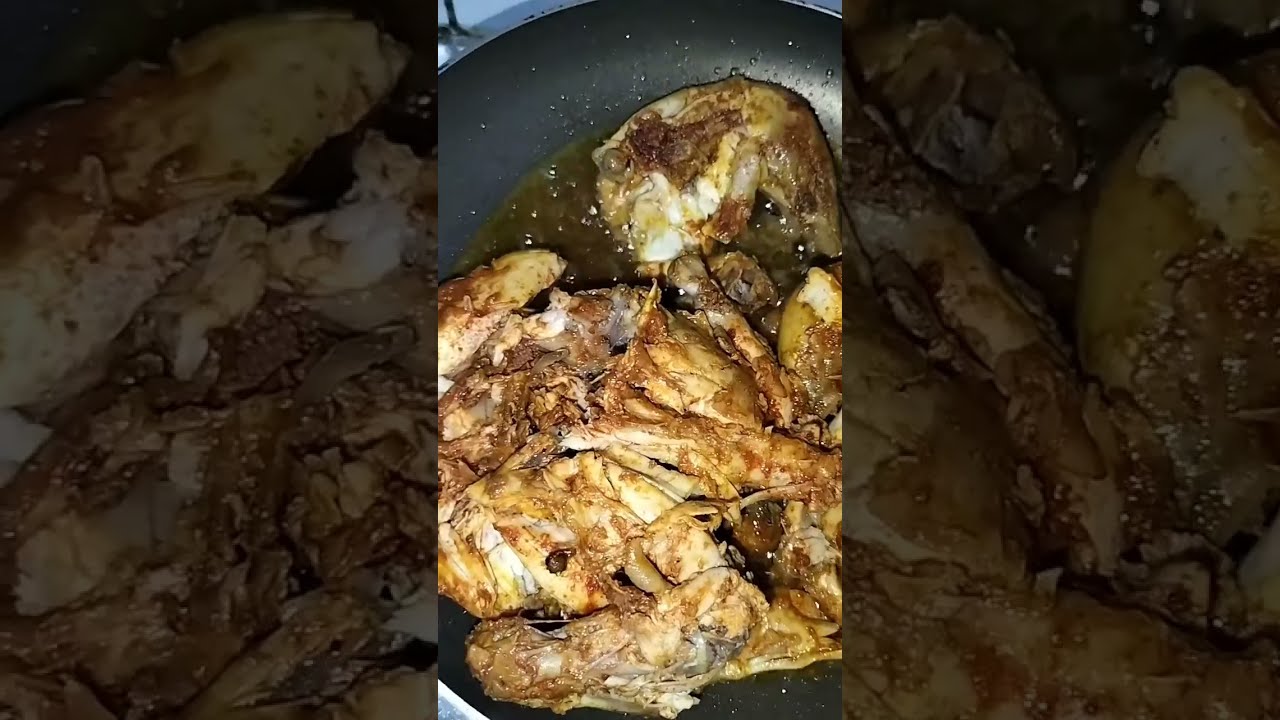The photograph captures an overhead view of meat cooking in a black, possibly nonstick frying pan. The image is taken in portrait orientation, and features mirrored, shadowed sidebars that extend it into a landscape format. Various cuts of meat, likely pork—though possibly chicken or organ meats—are sizzling and bubbling in a brownish, tannish juice. The meat appears well-cooked with brown and burnt markings, and is surrounded by shiny grease speckles and bubbling brown sauce. The pan's edges are cut off, focusing the viewer's attention on the center where the food is cooking. The scene is detailed with different shapes and sizes of meat pieces, sizzling with a rich, seasoned appearance.